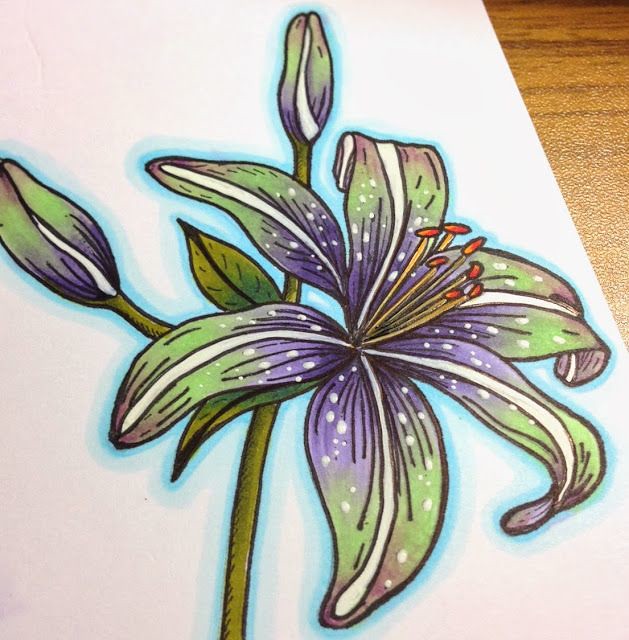The image showcases a brown wooden table upon which rests a light gray piece of paper. Centered on the paper is a striking flower with a vibrant green stem. The flower has five elongated petals that are predominantly purple and green, each adorned with a distinctive white stripe down the middle. The intricate details of the flower include brown stamens topped with bright orange tips. A lush green leaf extends from the stem, and nearby, there are two prominent buds with hints of white emerging, indicating they are on the verge of blossoming.